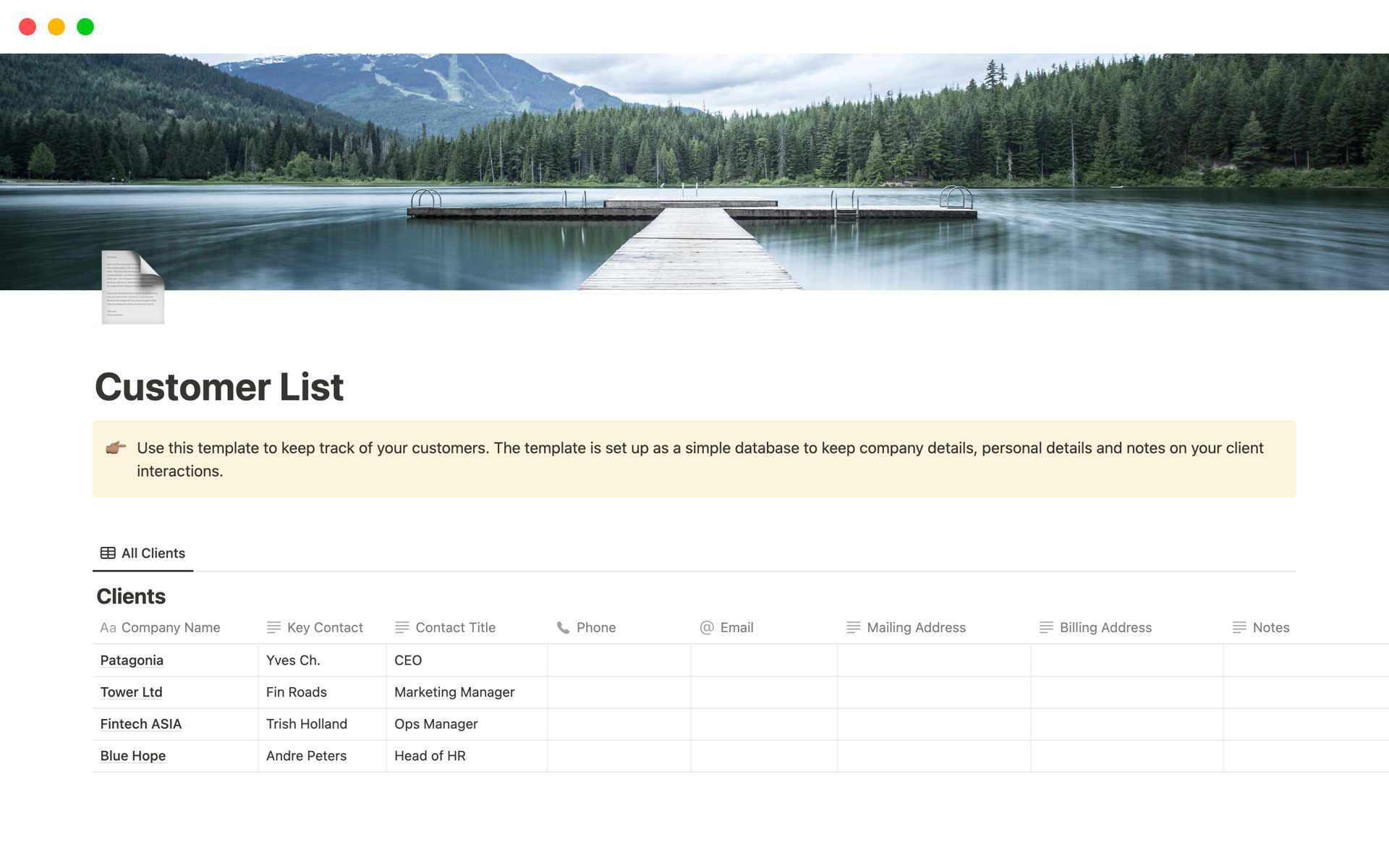This is a screenshot of a webpage titled "Customer List," spanning horizontally across the top of the screen. Dominating the visual space is a picturesque mountain and lake scene, where the lake occupies the foreground. Centrally positioned, a pier extends into the lake, forming a T-shape at its end. In the background, towering mountains are thickly blanketed with pine trees, while a few clouds linger in the distance, creating a serene and natural atmosphere.

Beneath this scenic photograph, the page transitions to a white background. Prominently displayed on this backdrop is the same "Customer List" header. Below this, a yellow or beige rectangular box stretches horizontally across the page. This box features an icon of a right-pointing finger, emphasizing instructional text that reads: "Use this template to keep track of your customers. The template is set up as a simple database to keep company details, personal details, and notes on your client interactions."

Following this instructional box, the page presents a detailed table designed for client information. The table includes multiple columns labeled: Company Name, Key Contact, Contact Title, Phone, Email, Mailing Address, Billing Address, and Notes. This structured format facilitates organized and efficient tracking of customer details.